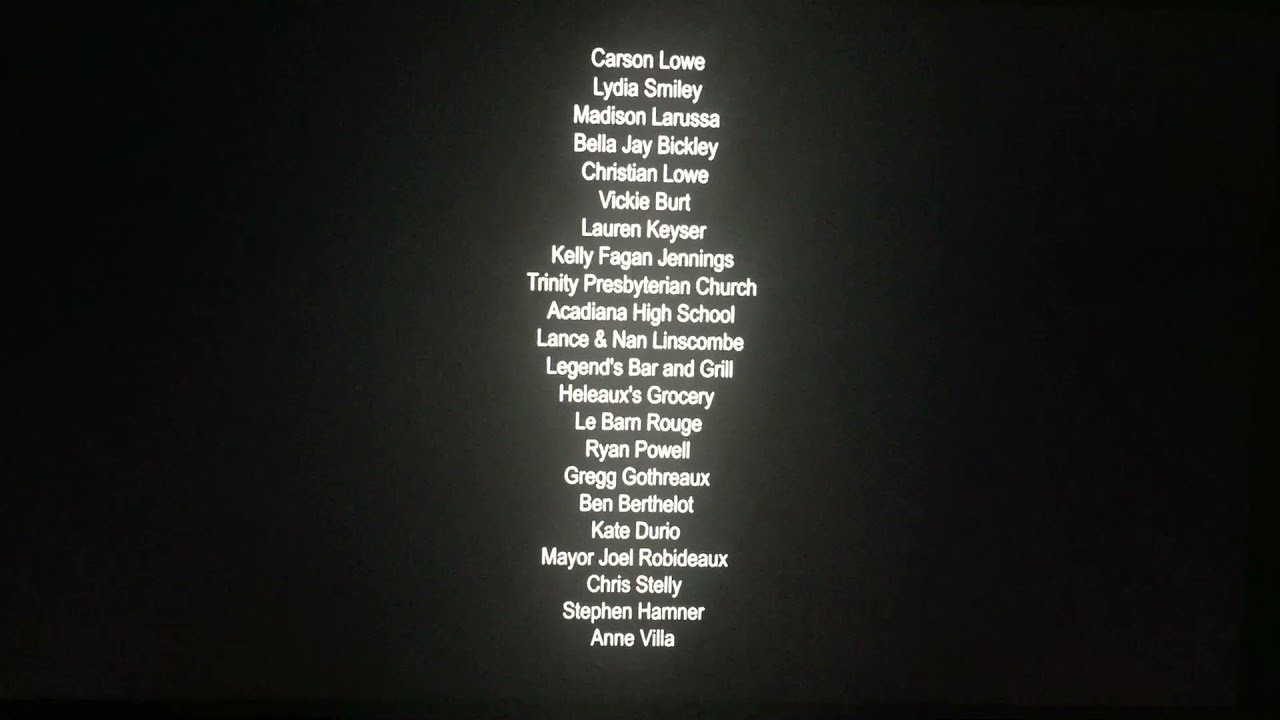The image depicts a wide rectangular black screen filled with a centered list of names and entities in white text, resembling closing credits from a movie. The text is slightly diffused with a glowing effect, suggesting it might have been photographed from a screen. The names, listed from top to bottom, include Carson Lowe, Lydia Smiley, Madison LaRussa, Bella J. Bickley, Christian Lowe, Vicki Burt, Lauren Kaiser, Kelly Fagan Jennings, Trinity Presbyterian Church, Acadiana High School, Lance and Nan Linscombe, Legends Bar and Grill, Hello's Grocery, Le Barne Rouge, Ryan Powell, Greg Gothro, Ben Berthelot, Kate Durio, Mayor Joel Robodeau, Chris Stelly, Stephan Hamner, and Ann Villa. The text stands alone in the center against a solid black background, reinforcing the impression of an end-credits roll or a similar acknowledgment list.